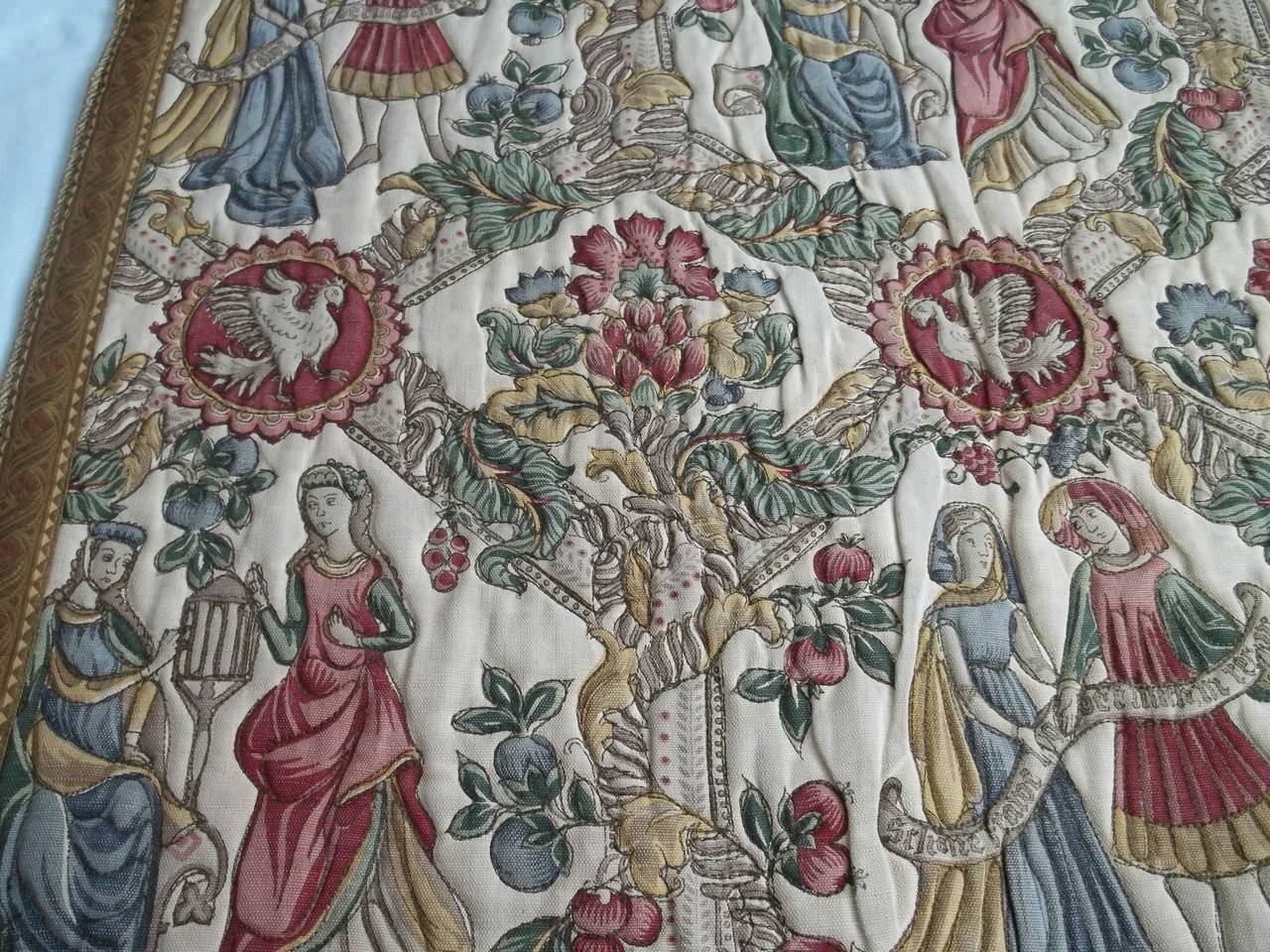This image showcases a richly detailed, possibly historical quilt or blanket, predominantly featuring intricate designs and a white background. At the bottom of the blanket, two individuals, one in a blue dress and the other in a red dress, stand side by side, seemingly engaging with each other while holding various objects. The middle section is abundant with plants, notably featuring apples, and is bordered by maroon circular designs. Each of these circles contains a bird; one faces left while the other faces right, creating a symmetrical, reflective pattern. The top of the quilt mirrors the bottom, depicting the same two individuals engaging in similar activities. Despite the overall white backdrop, the predominant colors used also include shades of light blue, red, pink, green, and yellow. The attire of the figures appears historical, reminiscent of fashion from the 15th to 18th centuries. Additional symbols, particularly the circular red ones with bird motifs, enhance the detailed visual narrative.